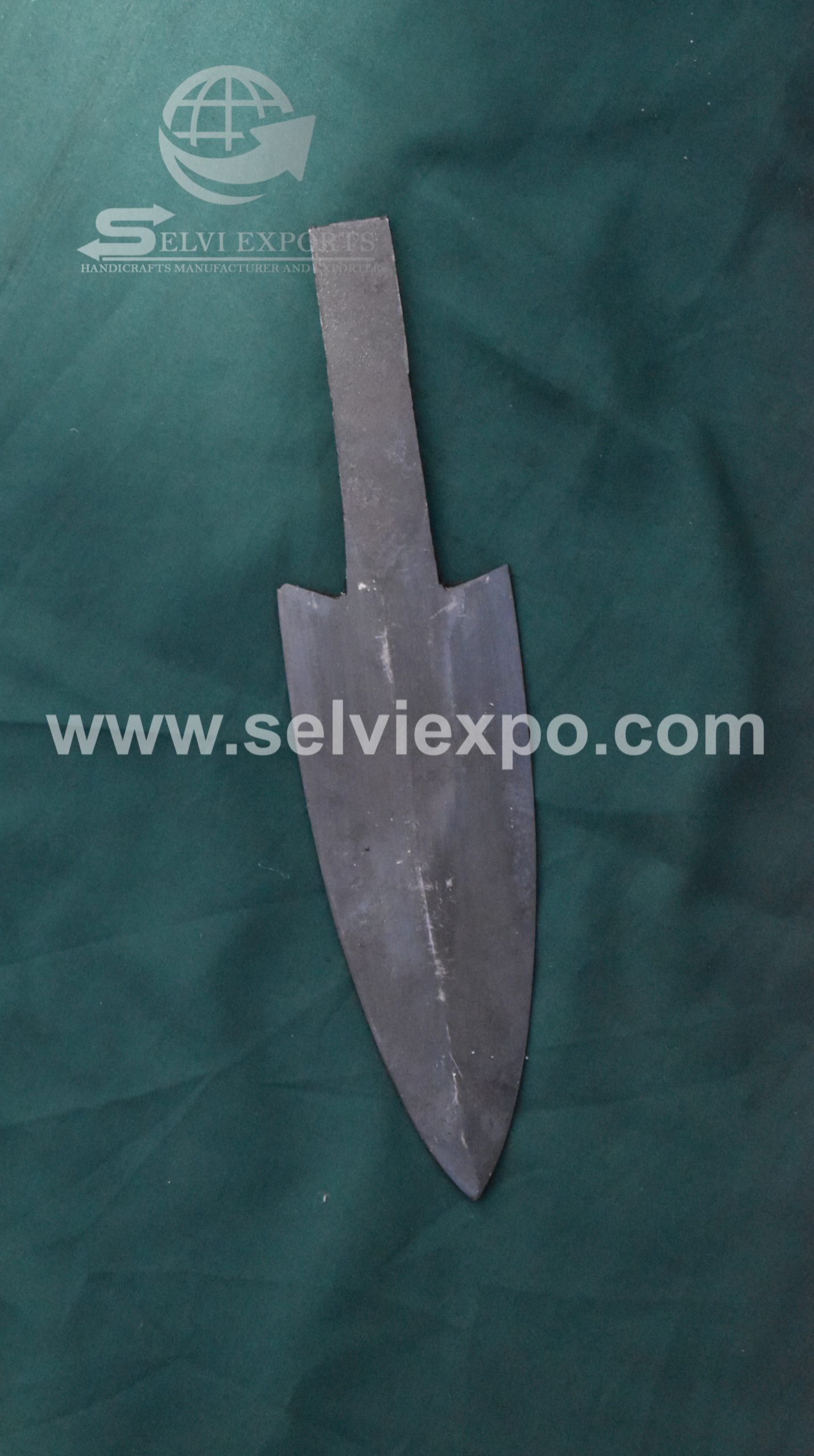This image depicts what appears to be a garden tool or a spear tip, prominently positioned in the center. The tool, made of metal and resembling either a small hand shovel or a spear tip, rests against a green jade-colored sheet, which serves as the backdrop for the display and is slightly wrinkled. The background features the website "www.selvyexpo.com" in white text, advertising the company's site. At the top of the image, there is a logo of a globe with an arrow pointing to the right, underneath which "Selvy Exports Handicrafts Manufactured and Exports" is written, suggesting the company's name and business focus on handcrafted items and exports. The overall presentation appears basic yet functional, aiming to advertise the company's products.